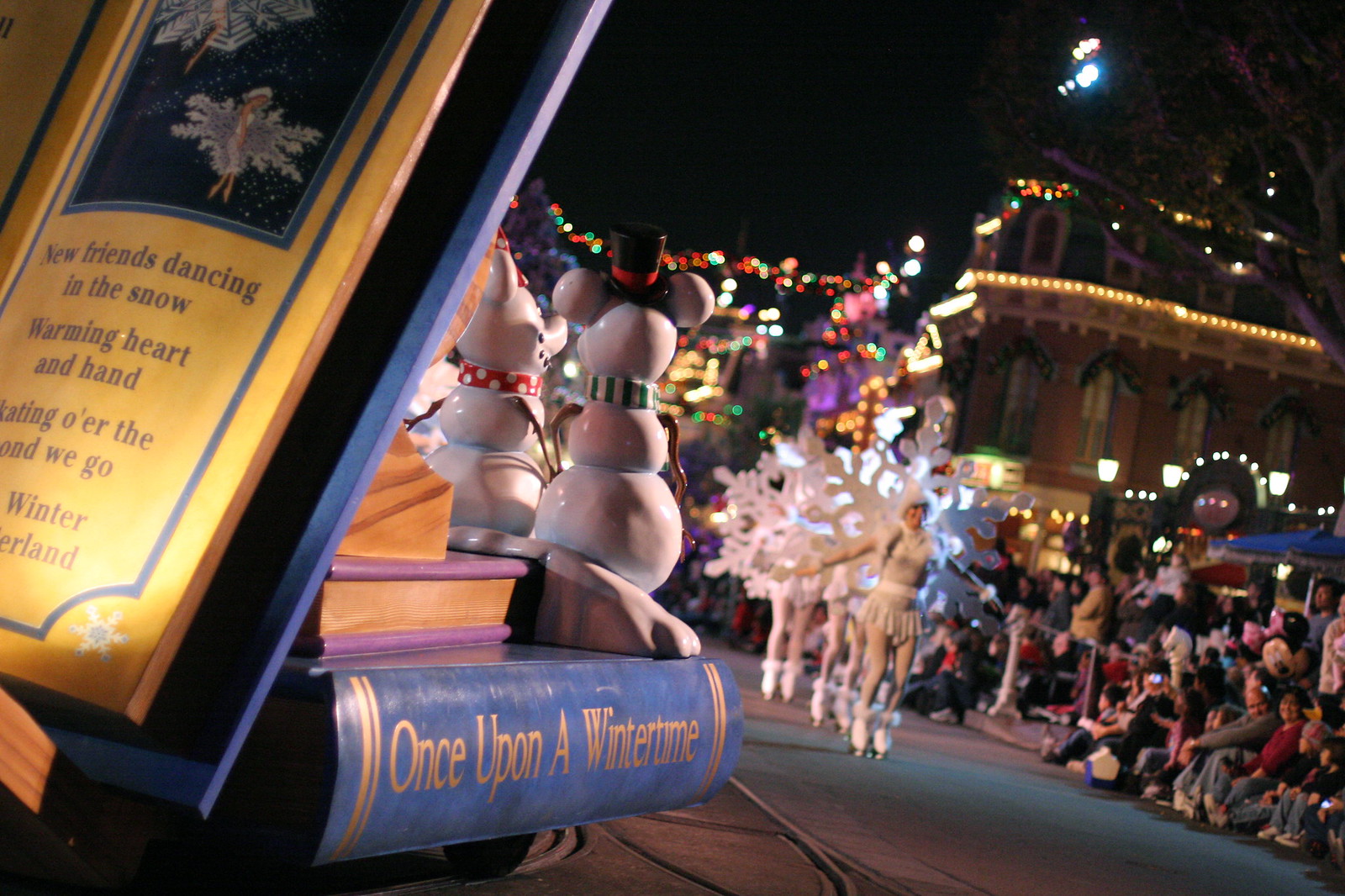The image captures a vibrant winter parade at night, blending the magic of storytelling and festive celebration in a single frame. On the left side, a close-up reveals an enchanting stack of books. The prominent blue-outlined open book reads, "New Friends Dancing in the Snow, Warming Heart and Hand," with some text cropped out below. Another book titled "Once Upon a Winter Time" lies in front, adorned with two snowmen, sticks for arms, and rounded mouse ears, adding a whimsical touch.

To the right, the street is alive with motion, where women in identical white skirts and skates, decorated with fur trim and large glowing snowflakes on their backs, gracefully glide on a strip of ice. Their outstretched arms create an elegant line against a backdrop of shimmering, multi-colored lights in hues of red, yellow, and green. A large crowd of children and families sits along the paved edge, watching in awe. The background buildings, festooned with holiday lights, blur into the dark night sky, while additional decorations and a lit tree add to the festive atmosphere. This color photograph in landscape orientation beautifully captures the essence of a winter wonderland brought to life through a nocturnal parade.